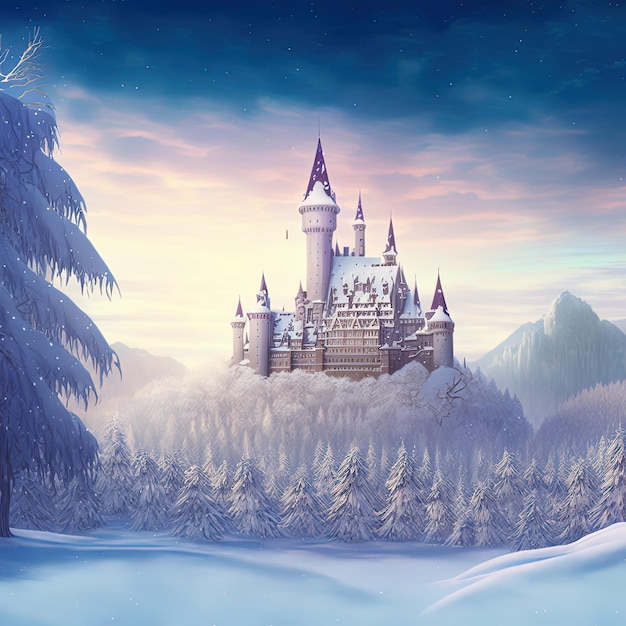In this enchanting, animated winter scene, a fairytale castle stands majestically atop a snow-laden hill, surrounded by a serene forest of snow-draped pine trees. The castle, positioned centrally, boasts eight pointed spires of varying sizes, with a prominent larger spire toward the left side. The steep, gray rooftops collect snow, giving the structure an ethereal appearance. Below and encircling the castle, a meadow covered in pristine, smooth, undulating snow stretches out, reflecting a soft blue hue. The landscape is framed on the left by a large snow-covered evergreen tree, its branches bending under the weight of the snow. The scene extends outward to encompass a row of pine trees, their shadows casting delicate patterns on the snowy ground. In the background, mountains rise on both sides of the castle beneath a sky that transitions from the dark of night, sparkling with stars, to the lighter shades of dusk, contributing to the magical, otherworldly atmosphere of the image.